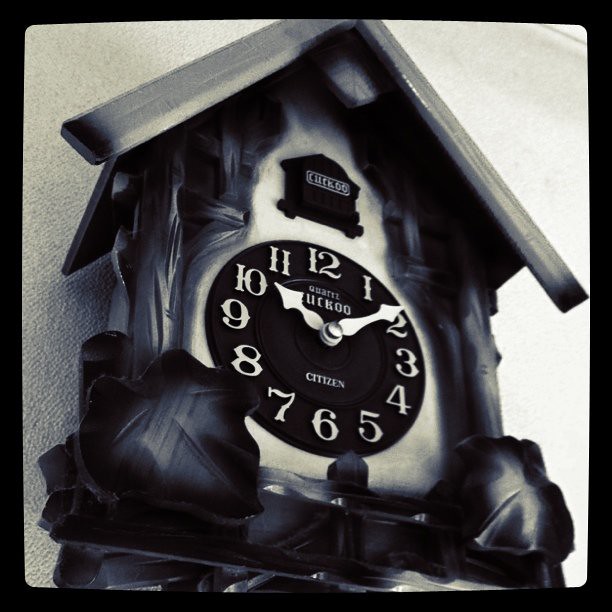This close-up photograph captures the intricate details of a wooden cuckoo clock from the perspective of someone standing directly beneath it and looking upwards. The clock, crafted entirely from wood, features an arched design resembling a birdhouse at the top and solid wooden sides. Each bottom corner is adorned with lifelike wooden leaves, displaying a charming gradient of color—lighter at the center and darker towards the edges, with delicate veining detailed through subtle grooves. The clock face is strikingly black, accentuated by white, raised numerals. The time is shown as 10:10 with stark white hour and minute hands. Above the clock face, a small black door awaits the cuckoo's appearance, marked with the word "Cuckoo" in white lettering. The front of the clock also prominently displays the word "Cuckoo" and the brand name "Citizen," bringing a blend of whimsical tradition and precise timekeeping to the piece.